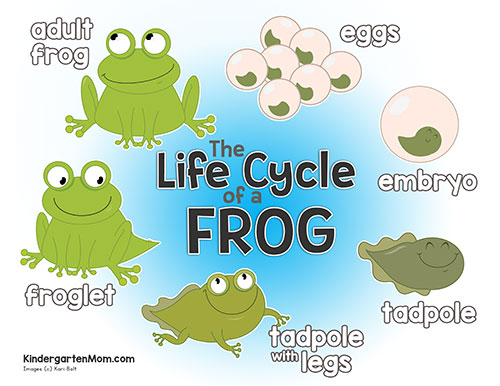This detailed infographic depicts the life cycle of a frog on a light to dark blue gradient circular background. At the center, the title "The Life Cycle of a Frog" is prominently displayed in cartoony text. Starting from the upper left, a lime green adult frog with circular eyes looks up and to the left, labeled "Adult Frog" in white text with a brown outline. To its right are frog eggs represented by light brown circles, each containing a green lima bean shape, labeled "Eggs." Moving further right is a large pink circle with a smiling green embryo inside, labeled "Embryo." Continuing downward, you find a dark green happy-faced tadpole labeled "Tadpole." At the six o'clock position is a lighter green tadpole with four legs, labeled "Tadpole with Legs." Finally, moving up and to the left is a froglet with a pointy tail and a smile, labeled "Froglet." Each stage is depicted in a cartoon style with emphasis on the smiling faces. The bottom left corner features small black text, "kindergartenmom.com," denoting the source of the infographic.